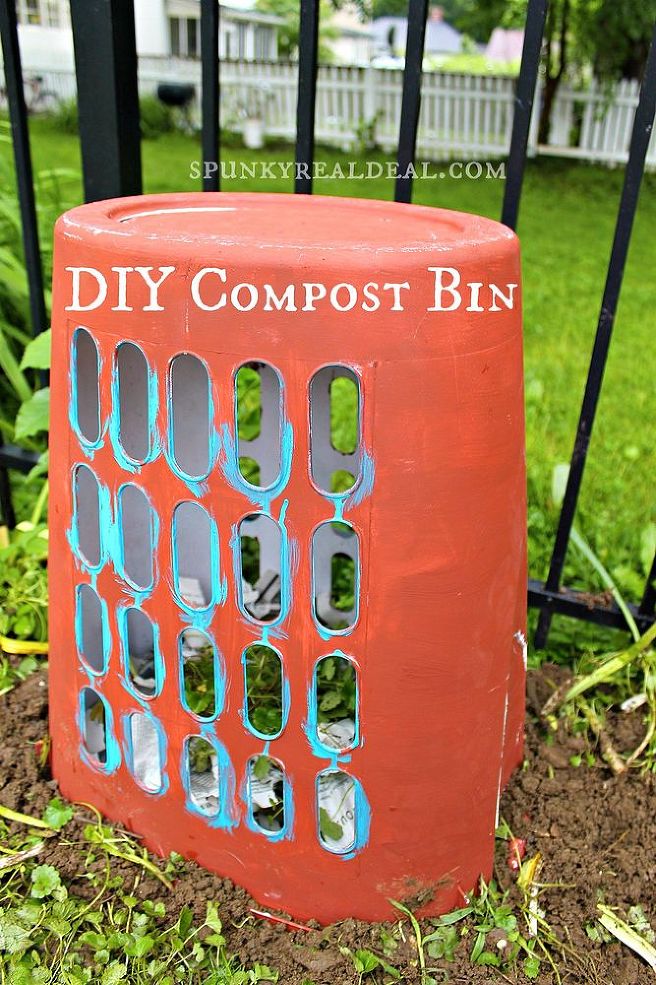In this vivid outdoor photograph, a brightly colored orange-red DIY compost bin, fashioned from a plastic laundry basket with oval-shaped openings on the sides, occupies center stage. The bin, positioned upside down with the base facing up, prominently displays the label "DIY Compost Bin" in white letters along with the website "spunkyraildeal.com." The orange paint on the bin appears to be chipping, revealing traces of blue paint beneath it. Inside the bin's base, some herbs or weeds are visible, though it is far from full. The bin is set on the earth, surrounded by sparse dirt, grass, and leaves. In the background stands a see-through black metal fence, beyond which a lush green lawn, a white wooden fence, parts of a white house, and what seems to be a grill are seen, adding context to the garden setting.